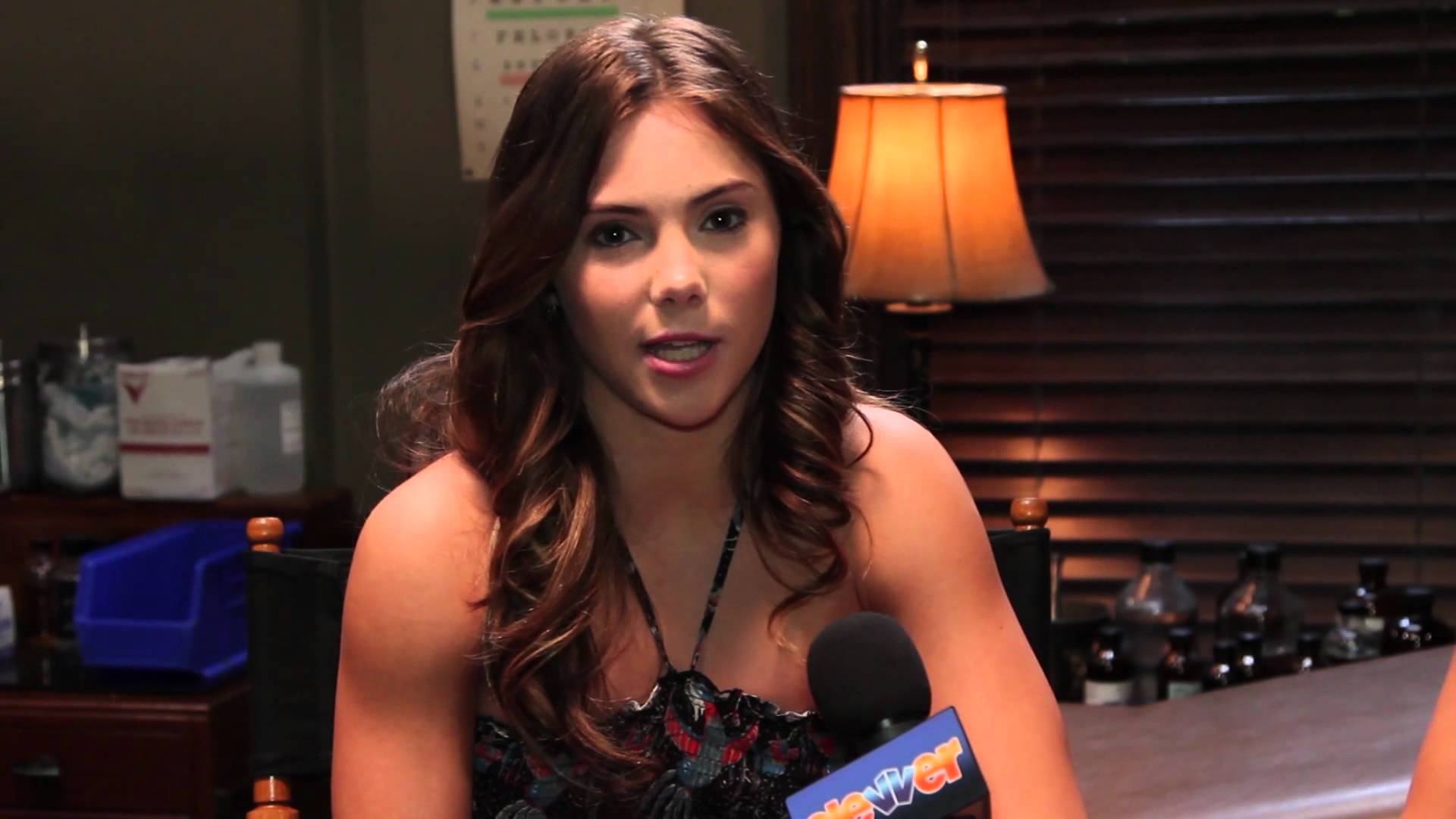In this detailed photograph, a young Hispanic woman, likely in her early twenties, is captured mid-action, possibly as a news reporter or speaker. She has long, curled brown hair and dark brown eyes. Her facial features are delicate, enhanced by a light application of blush and light pink lipstick. Her attire consists of a dress with thin straps that feature a vibrant red flowery design, leaving her shoulders bare.

She is holding a microphone near her chest, slightly cut off in the image. The microphone has a foam windscreen and a boxy base displaying partially visible text, with the letters "ELE," "VV," and "ER" in a mix of orange and blue colors, suggesting it might spell out "DEVVER" or something similar.

The background includes a variety of items: a glowing lamp emitting an orange hue, partially visible blinds, and indistinguishable shapes that might be bottles of water or bins. The setting appears to be indoors with a mixture of colors dominating the scene, including yellow, orange, tan, brown, blue, and red. The presence of these elements along with the indoor indicators like the lamp and blinds points to an indoor setting, although the time of day is indeterminate.